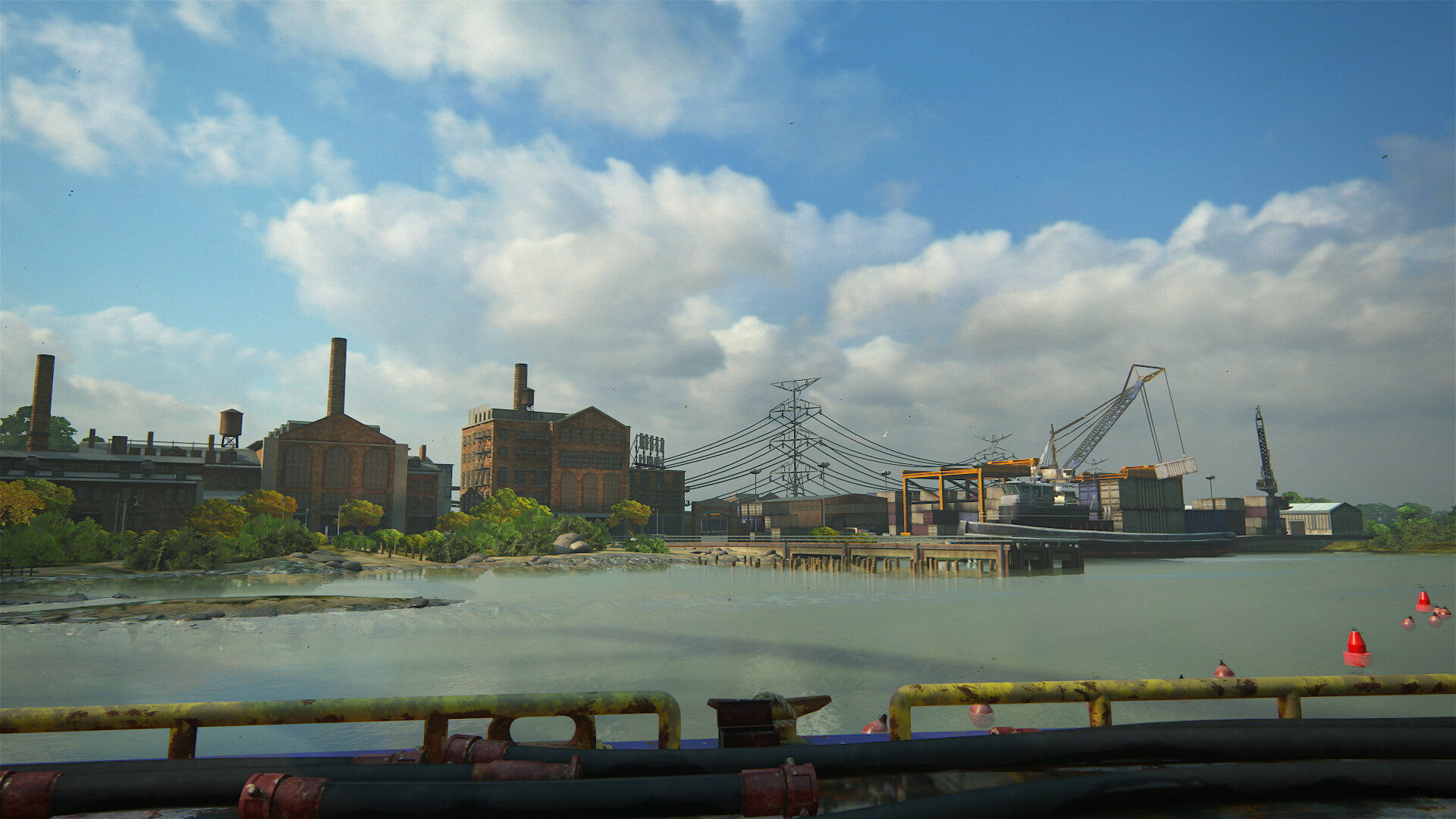The image captures a detailed industrial waterfront scene, likely taken from a dock or a boat. In the foreground, the dock is characterized by a yellow edge with a cleat for securing an anchor rope and some yellow railings. A set of large hoses with couplings, resembling fire hoses, are also noticeable. The water, with an unusual green tint suggesting algae, features several red buoys—ranging from five to eight. 

Extending from the docks are views of a sprawling industrial landscape across the water. This area includes three prominent orange brick warehouses with long smokestacks, though no smoke is visible currently. Additional industrial elements, like a crane positioned to the right, numerous telephone wires and electrical lines, highlight the utilitarian nature of the environment. 

A structure juts out into the water from the center of the scene, adjacent to which are patches of greenery including trees and bushes lining the left and right edges of the waterway. These natural elements contrast with the industrial atmosphere. 

Above, the sky stands out in stark blue, adorned with large, billowy white clouds, giving the overall scene a picturesque quality despite its industrial setting.